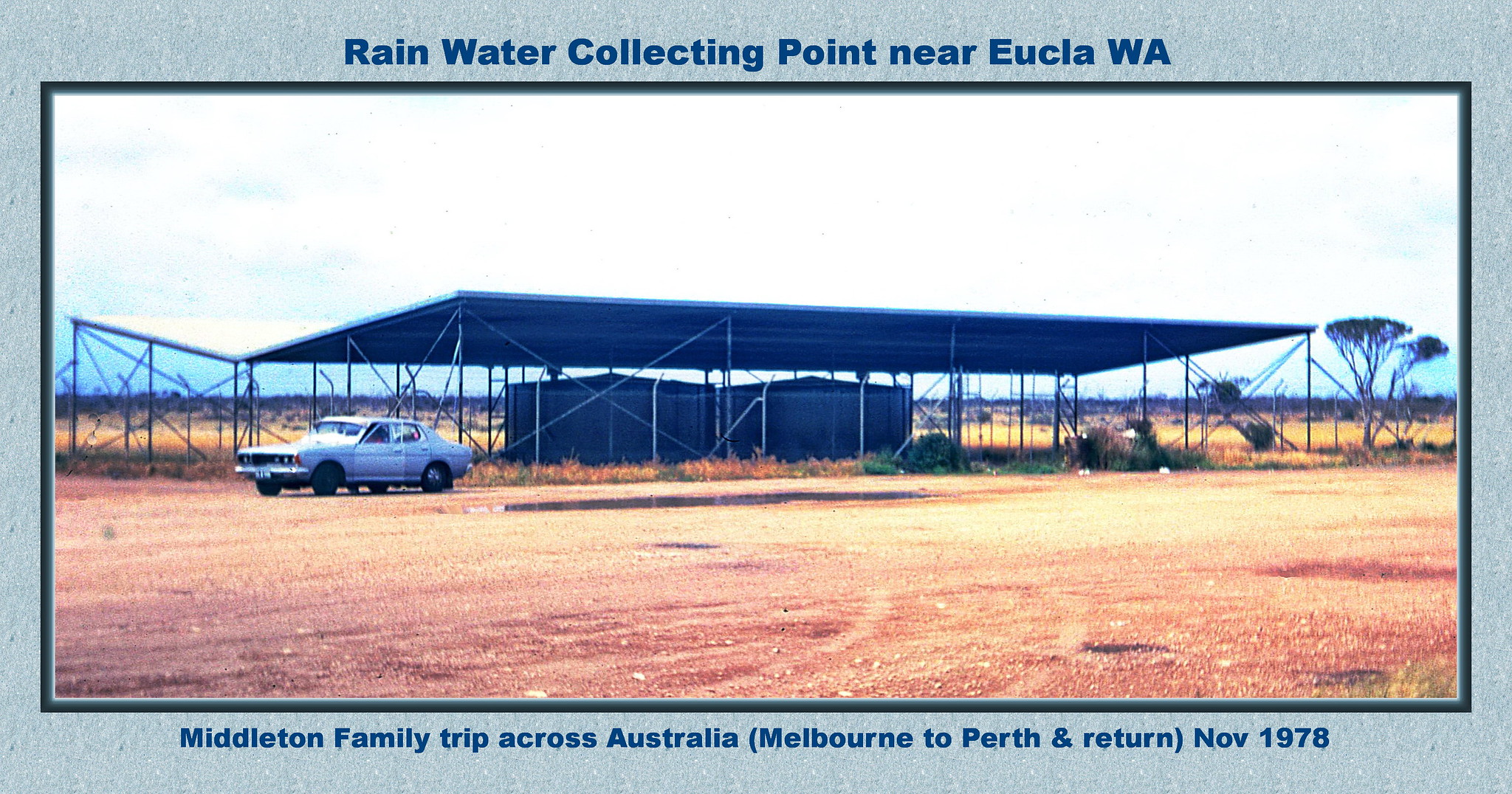The vintage photograph, bordered by a light blue and dark blue frame, captures a scene from the Middleton Family Trip across Australia, spanning Melbourne to Perth and return in November 1976. Titled "Rainwater Collecting Point near Eucla WA," the image shows an outdoor structure in a desolate field. The foreground features a brown, sandy road, while the background reveals a gray, cloud-laden sky. Dominating the scene are two large, dark cylindrical basins, likely grey or black, designed for rainwater collection and sheltered by a slanted roof supported by a trellis. To the left, a vintage four-door sedan is parked, adding to the snapshot's nostalgic feel. Sparse vegetation, including short, leafless trees, dot the barren landscape, underscoring the arid and unwelcoming environment typical of the Australian outback.